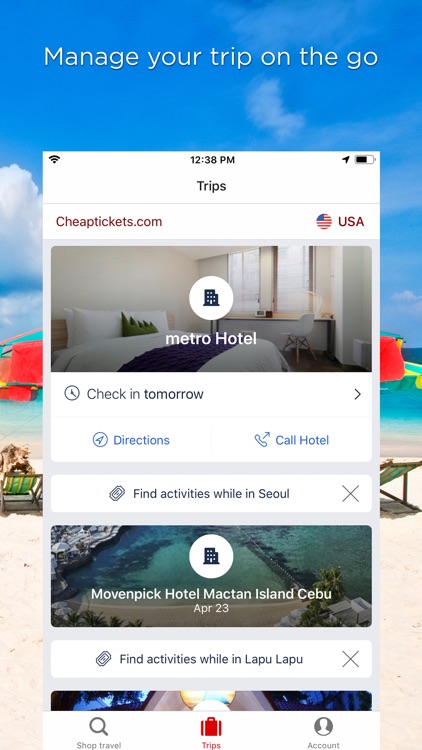The image is a promotional screenshot from CheapTickets.com. The background features a vibrant and tropical beach scene, complete with beach cabanas set against a clear, azure sky dotted with fluffy white clouds. 

At the very top, large text reads “Manage your trip on the go.” Superimposed onto this scenic backdrop, a smartphone screenshot displays the CheapTickets app in use. 

At the top of the phone’s screen, the app's interface shows “Trips” along with the CheapTickets.com logo on the left and “USA” on the right. Below this, there’s a photograph of a hotel room with “Metro Hotel” written prominently in white font. Above the hotel's name, a white circle contains an icon of a building. Just below the hotel name, the text reads “Check-in tomorrow” followed by options for “Directions” and “Call hotel.” 

Further down, a small box with a link instructs users to “Find activities while in Seoul,” spelled out clearly. 

A large "X" button is present below this section, suggestive of an option to close the screen. Beneath this button, another photograph appears with the text “Movenpick Hotel, Mactan Island, Cebu.” Below this, the same functional link invites users to “Find activities while in Lapu-Lapu.”

At the very bottom of the onscreen display, navigation buttons labeled “Shop,” “Travel,” “Trips,” and “Account” are visible.